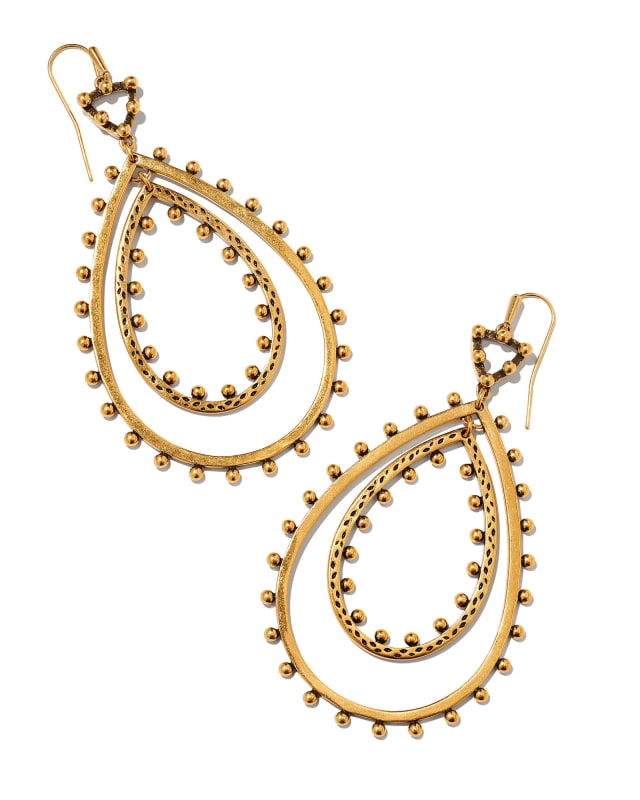In this detailed color photograph, there are two matching pieces of gold-colored jewelry, appearing to be earrings possibly made out of brass or with a wood-like tan gold finish. The earrings are large hoops designed with a single hook at the top, which arches to stay in the ear. The top of each earring features a triangular shape, which transitions into two concentric, almond or eye-shaped ovals. These ovals are adorned with numerous small gold beads, meticulously attached both inside the smaller oval and around the external perimeter of the larger oval. Intricate artwork embellishes the central gold piece, enhancing the unique and eye-catching design of these earrings.